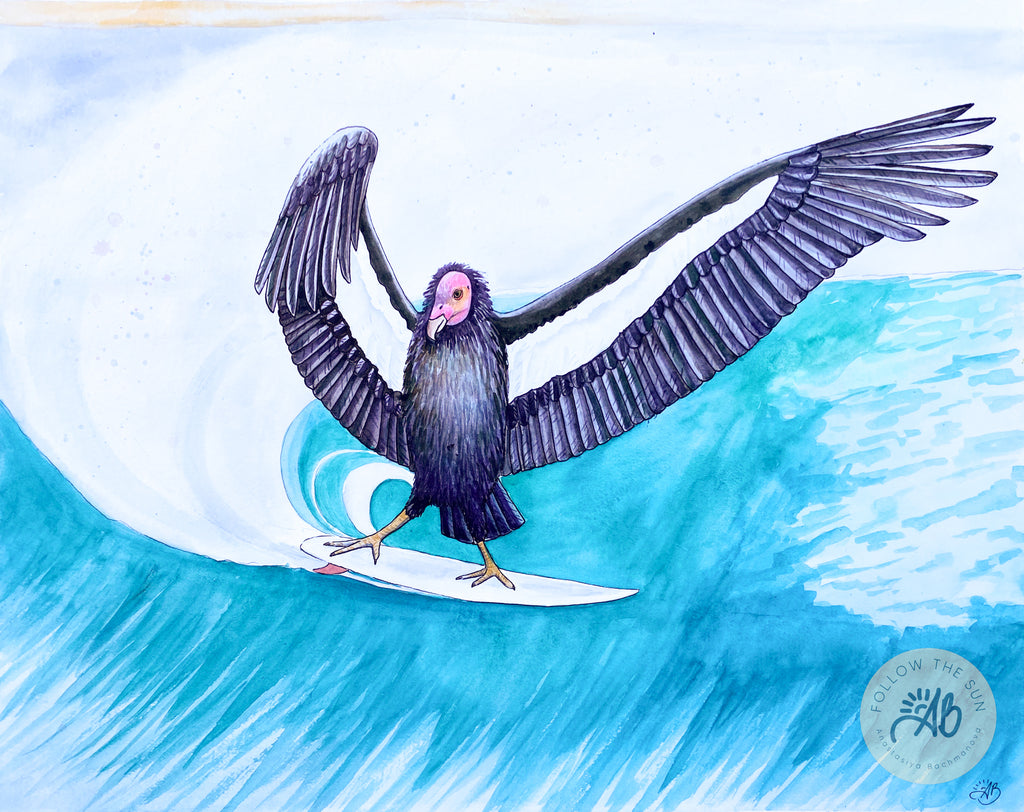The image is a detailed and vibrant drawing of a cartoon bird riding a surfboard on the ocean. The bird, which has the body of a black raven and a head resembling that of a vulture or skeleton, features a pink, featherless face with a white beak and a single, wide-open yellow eye. Its extensive, layered wings are spread wide as it balances on a white surfboard with a red fin. The bird's small yellow legs and three-toed feet are positioned to maintain balance. The ocean, depicted in various shades of blue with darker tones at the bottom, showcases artistic wave patterns highlighted by white strokes. A large wave caps in white and fades into a white sky, covering the top half of the image. Additionally, in the bottom right corner, there is a text and logo reading "Follow the Sun" with the initials "AB," presumably the artist's signature.